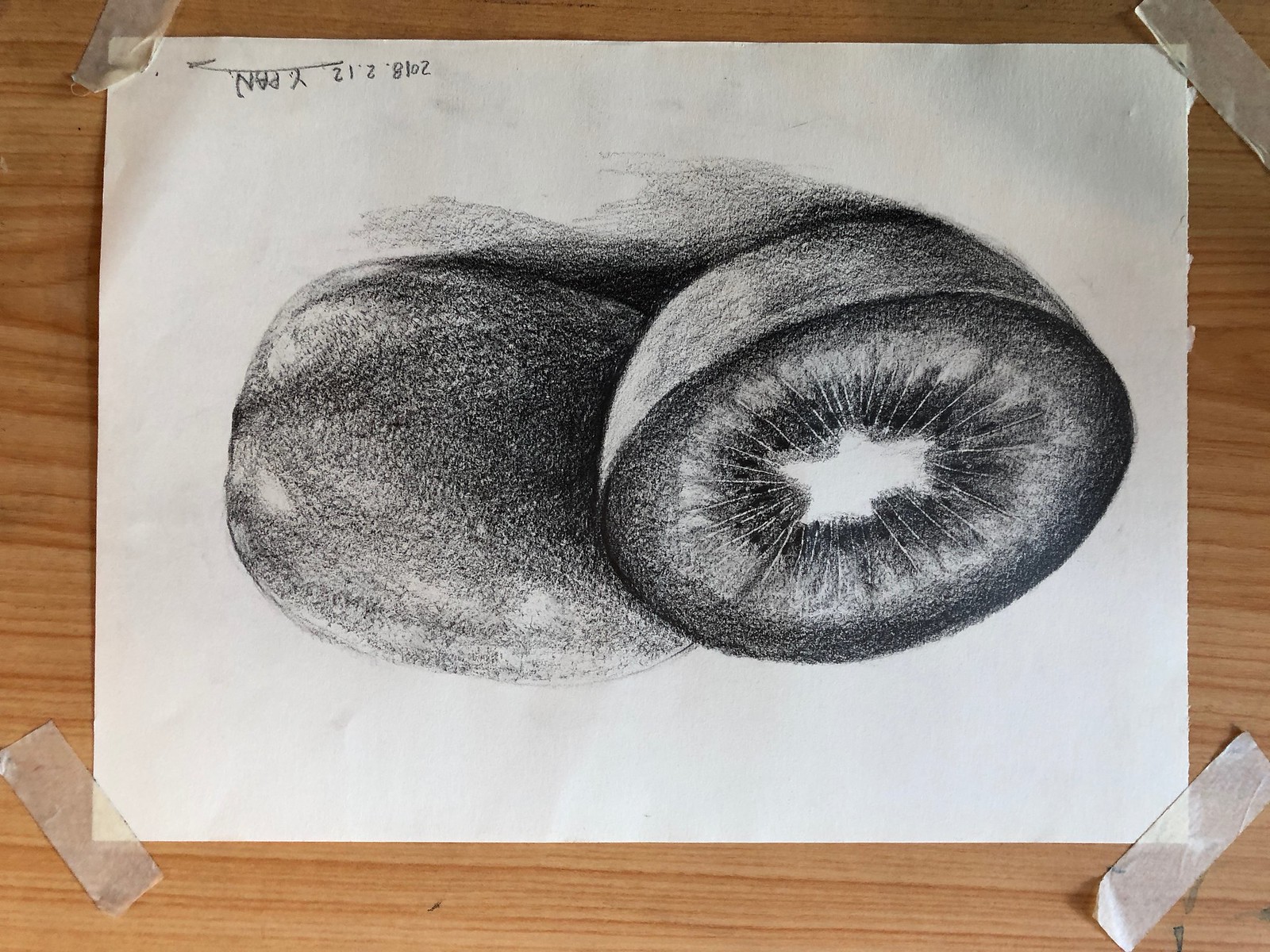This intricate sketch depicts two kiwis on a sheet of paper: one whole and uncut, showcasing its fuzzy, oval exterior, and one sliced in half, revealing the fruit's vibrant center with seeds. The entire drawing is presented inverted at a 180-degree angle, creating a unique, upside-down perspective. The paper is taped to a wooden table or background with four pieces of tape, one on each corner, clearly visible and securing the artwork in place. The texture of the wooden surface provides a natural, rustic contrast to the detailed fruit sketch.